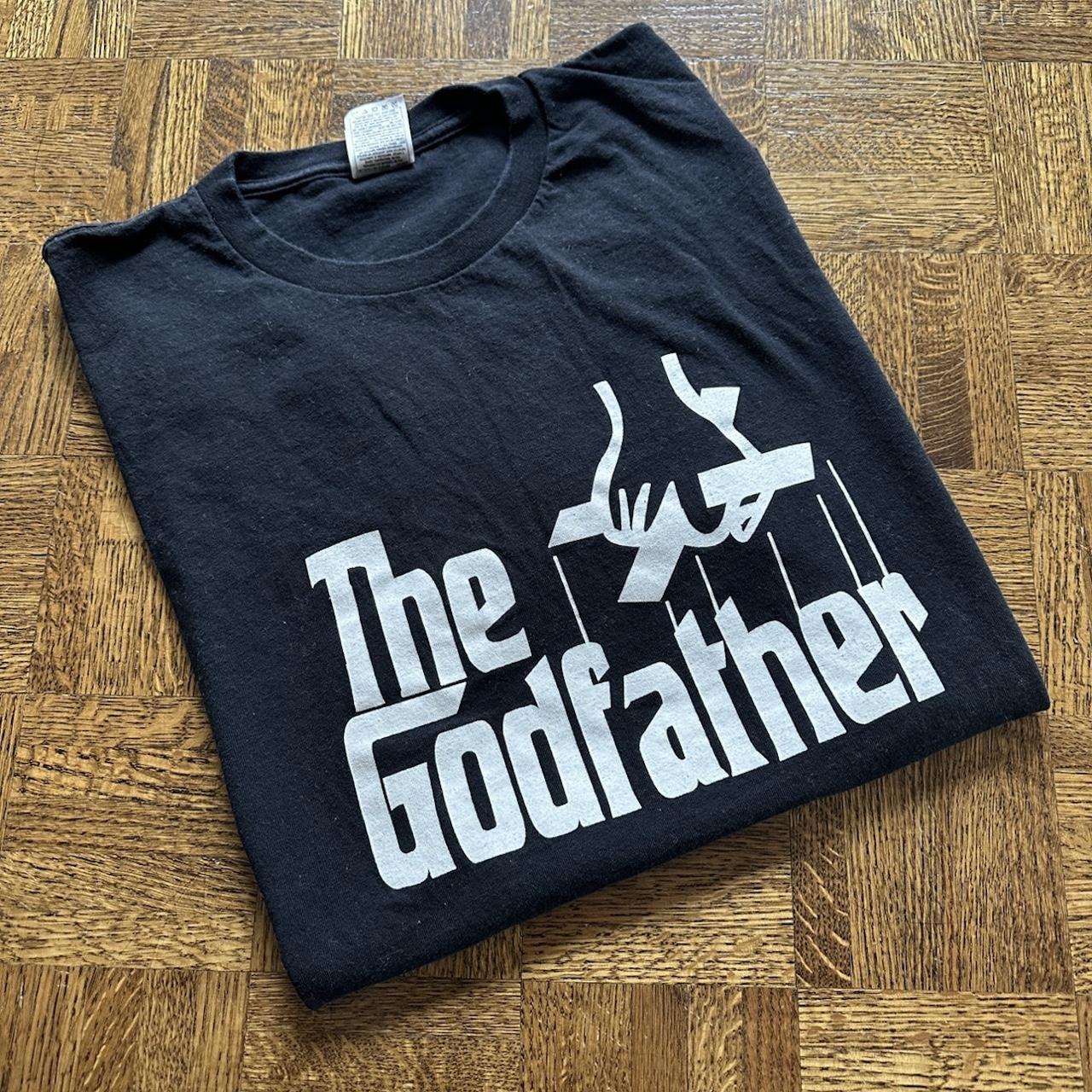This detailed close-up color photograph captures a neatly folded black t-shirt positioned slightly at an angle on a surface that appears to be made of wooden or faux wooden tiles with a distinct square pattern of alternating dark and light brown hues. Prominently displayed on the t-shirt in bold white lettering are the words "The Godfather," with both "T" and "G" capitalized. Above the word "father," a stylized black hand is depicted holding a cross-like wooden control, complete with strings leading down to the letters "F," "T," "H," "E," and "R," evoking imagery of puppeteering or manipulation. A small white tag is visible in the v-neck of the shirt, which is impeccably folded with subtle creases around the hand graphic, and dominates the composition, filling most of the image.